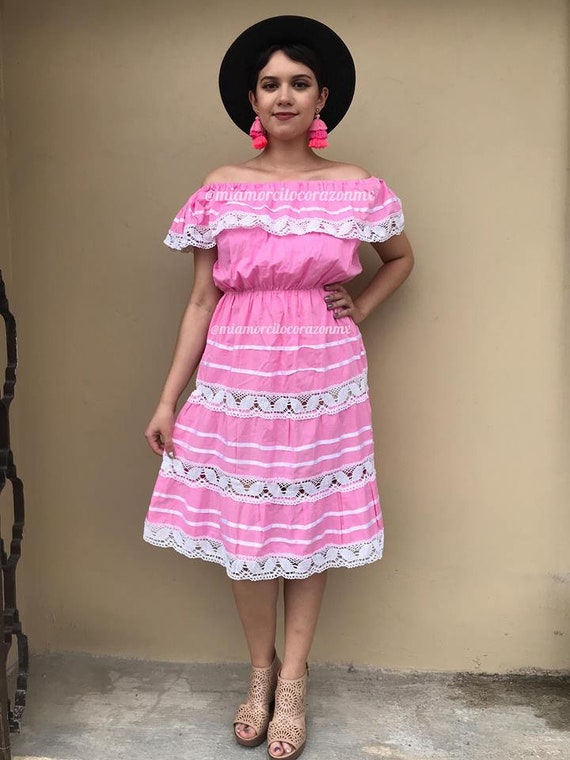In the outdoor photograph, a young woman with a nice tan is standing against a beige wall on a concrete floor, fully engaging the viewer with her poised stance and confident smile. She dons a light pink, off-the-shoulder, knee-length dress that features a high elastic waist and a flowing skirt. The dress is adorned with delicate white lace embroidery and regular white stripes. Her ensemble is accentuated by a wide-brimmed black hat that shades her dark, sleek hair, and large pink tassel earrings that add a playful touch. The woman complements her look with dark-colored lipstick and tan, open-toed wedge sandals, which give her a modest height boost. Her left hand is propped on her hip, while her right hand elegantly lifts the skirt of her dress to the side, showcasing its fullness. This color photograph, oriented in portrait, captures the essence of fashion photography with a touch of representational realism.